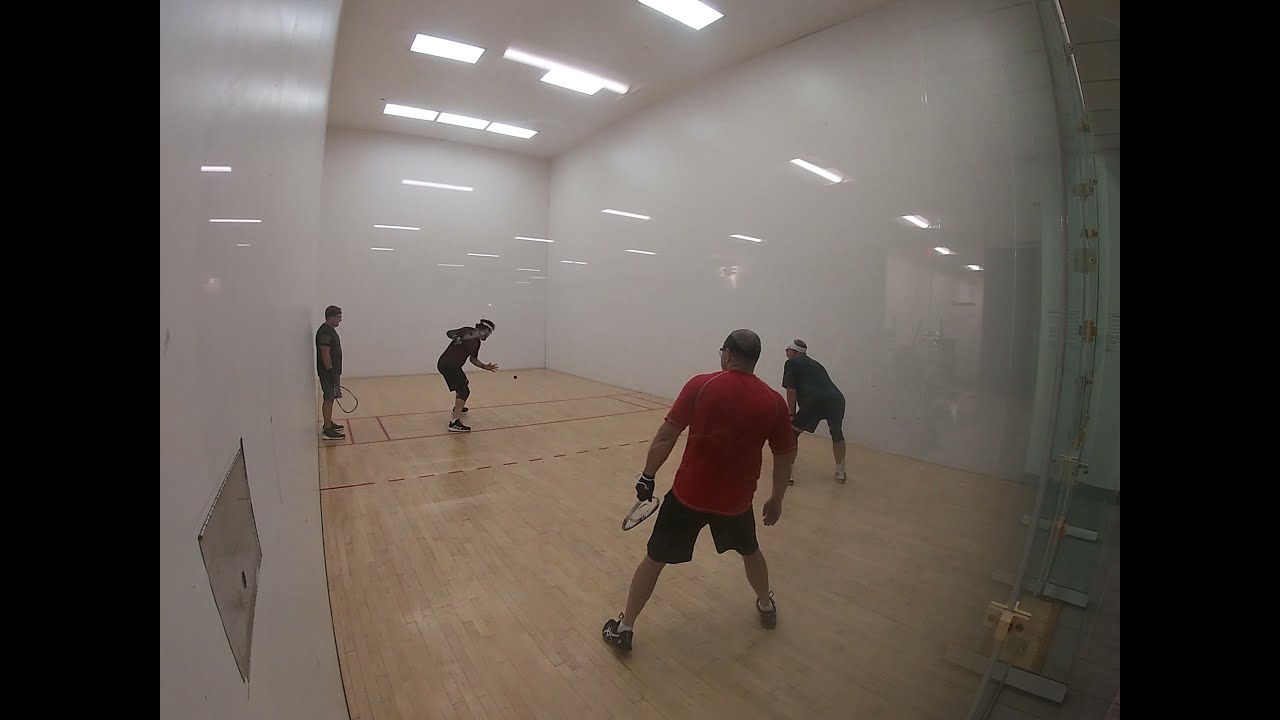In this detailed image of a racquetball game, four men are engaged in play inside an enclosed racquetball court with three pristine white walls and a reflective wooden floor. The room is well-lit with lights in the ceiling and reflections visible on the walls, creating a bright atmosphere. The back wall is made of clear plexiglass, allowing an external view into the court. 

In the foreground, a man dressed in a red shirt and black shorts is facing away from the camera, ready with his racquet and poised in tennis shoes. To his right, another player in a blue shirt, black shorts, and a headband is slightly crouched, preparing to respond to the ball that hovers in the air nearby. 

Across the court, on the left side of a floor marking that separates the players, a man in dark clothing is leaned over, seemingly about to serve the ball. Next to him, another player, also in dark-colored attire, stands against the wall observing the server with his racquet in hand. The scene is framed with the glass partition capturing reflections of external light, adding depth to the indoor setting.